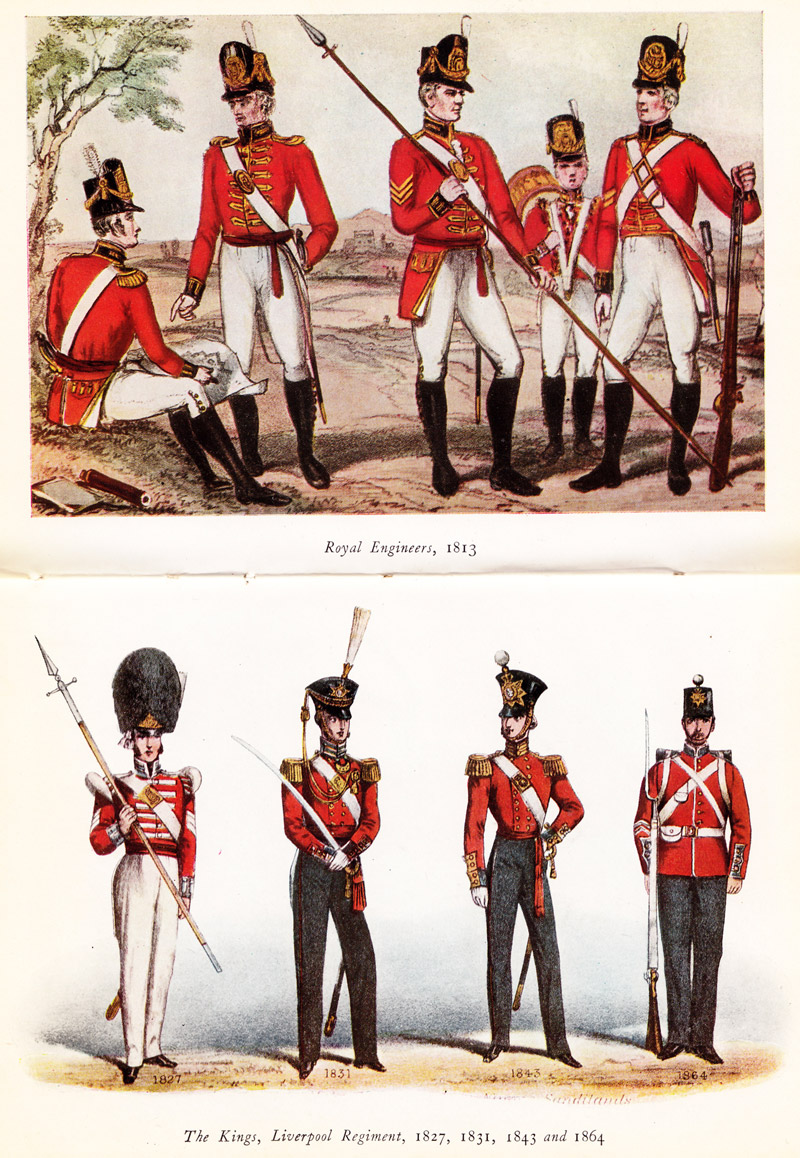The rectangular artwork, approximately six inches high and three to four inches wide, features two historical postcards arranged vertically. Each postcard, depicting English soldiers, tells a distinct story through their detailed uniforms and labels.

The top postcard, framed by a light border, is titled "Royal Engineers 1813" in black print at the bottom center. It showcases five men, one notably shorter and appearing younger, all clad in matching dark knee-high boots, white breeches, red long-sleeved coats adorned with black lapels, and tall black hats embellished with gold emblems and ribbons. Some wear white sashes, with one notably bearing two crisscrossing sashes. Their equipment varies—a sword, a musket, a spear, and a drum, indicating roles within the regiment.

Beneath this, the second postcard stands against a white background, labeled "The King's Liverpool Regiment 1827, 1831, 1843, 1864," illustrating the evolution of their uniforms across these years. The leftmost soldier, representing 1827, wears a substantial rounded black bear fur hat, a red long-sleeved tunic with white shoulder pads and horizontal straps, long white breeches, and small black boots, holding a spear. The subsequent figures, depicting later years, wear similar red tunics now paired with long black pants and black boots. The 1831 and 1843 soldiers feature tucked-in red shirts and gold shoulder pads, with black hats adorned with white feathers or balls. The 1864 soldier's uniform is notable for a longer, untucked red tunic with a white belt and crisscross strap, a black backpack with white straps, and a short black hat with a white ball on top, completing his look with a lengthy musket.

Set against a white background, this intricate illustration captures the historical attire of English soldiers, evocative of nutcracker figures often associated with Christmas, each element meticulously detailed to reflect their era and rank.